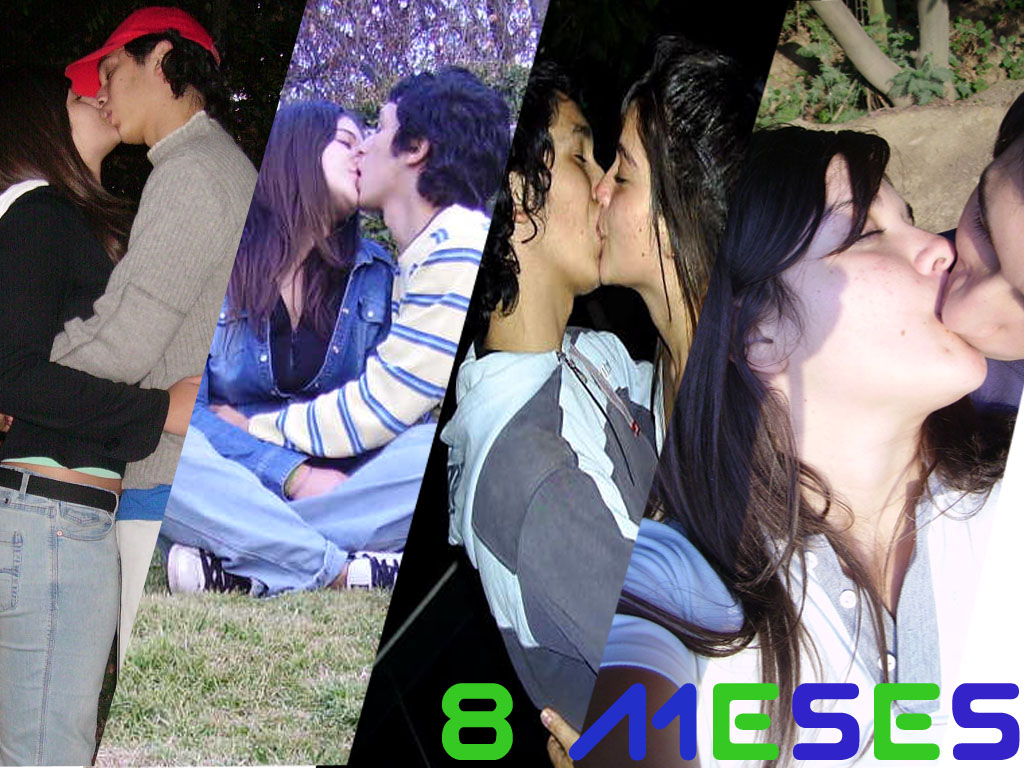A collage of four photographs captures the romantic moments of a young couple over what appears to be eight months, as indicated by the "8 meses" text in a futuristic green, blue, and purple computer-style font at the bottom. Each of the four images, arranged in a diagonal strip from lower left to upper right, showcases the couple kissing passionately in various settings and outfits. 

In the first image, the couple stands and embraces, with the young man wearing a red hat, grey sweatshirt, and white trousers, while the woman dons blue jeans and a black top. Both have brown hair and fair skin. 

The second photo depicts them in an outdoor scene, sitting on the ground and hugging, with the man dressed in a blue and white striped shirt and the woman in double denim—a jean jacket over a blue top, denim pants, and white trainers with black laces. 

The third image, a tighter close-up, shows the couple kissing again, with the man now wearing a light and dark blue hoodie. The woman's clothes aren’t fully visible, but she remains an integral part of this intimate moment.

In the final close-up photo, the woman, now on the left side again, can be seen more clearly, while the man's presence is mostly hinted through his brown hair and partial view. The backdrop suggests a natural, outdoor setting with glimpses of trees and sunlight.

The series collectively narrates a tale of young love, capturing both tender embraces and passionate kisses in varied contexts.